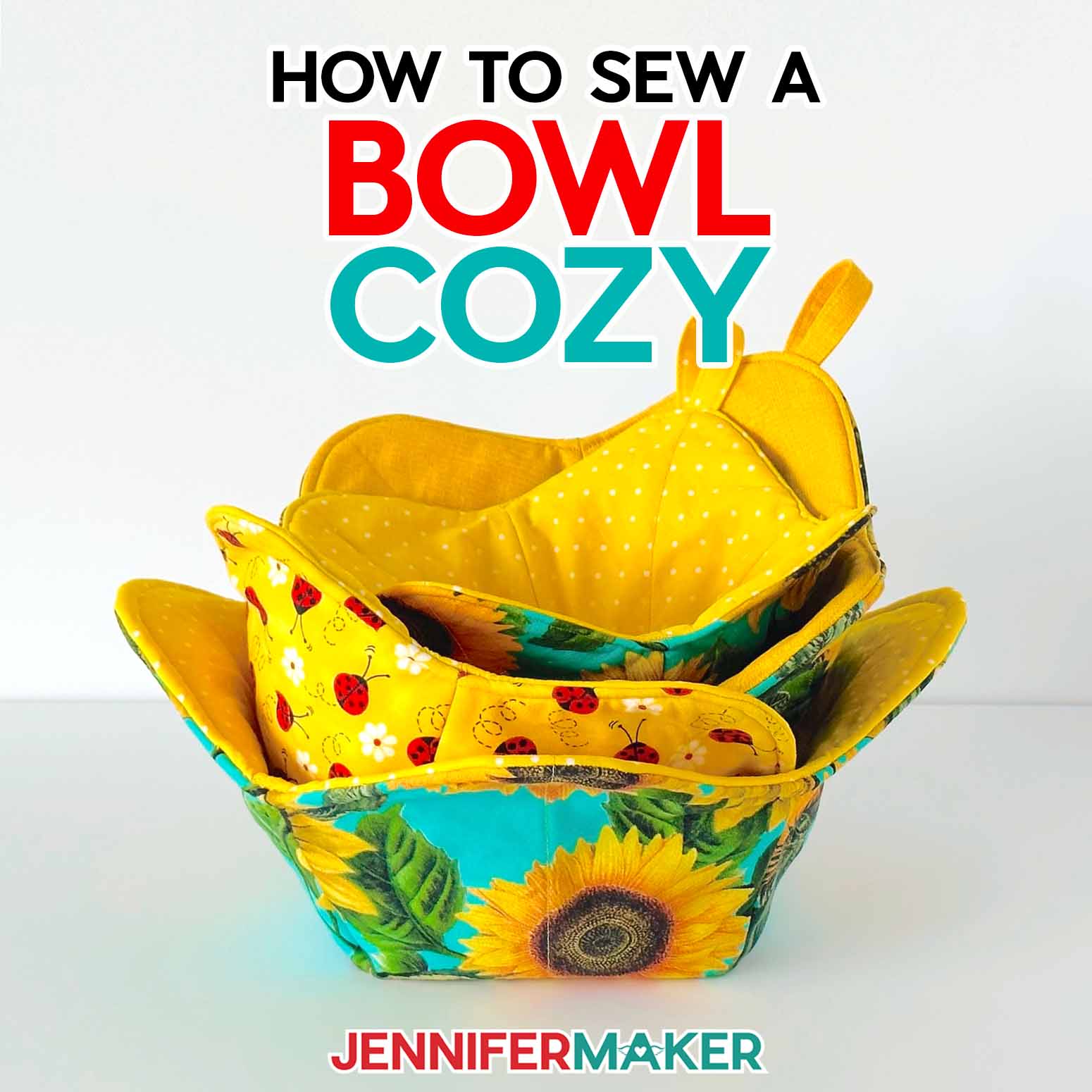The image depicts a book cover titled "How to Sew a Bowl Cozy." The title is prominently displayed in black text for "How to Sew A," and in red and blue text for "Bowl Cozy," with a unique heart-shaped 'A'. The author's name, Jennifer Maker, appears at the bottom with "Jennifer" in red and "Maker" in blue. This title appears on a plain white wall above a white table surface.

On the table, there is a stack of bowl cozies made from different patterned fabrics. The largest bowl cozy at the bottom of the stack is adorned with big yellow sunflowers and green leaves. Inside this, there are more sunflower-patterned bowl cozies and one featuring a yellow fabric with red ladybugs and white flowers. The inner surface of the outermost bowl cozy is a bright yellow with white polka dots. All these fabric bowls fit neatly within each other, offering a mix of vibrant and cheerful designs.